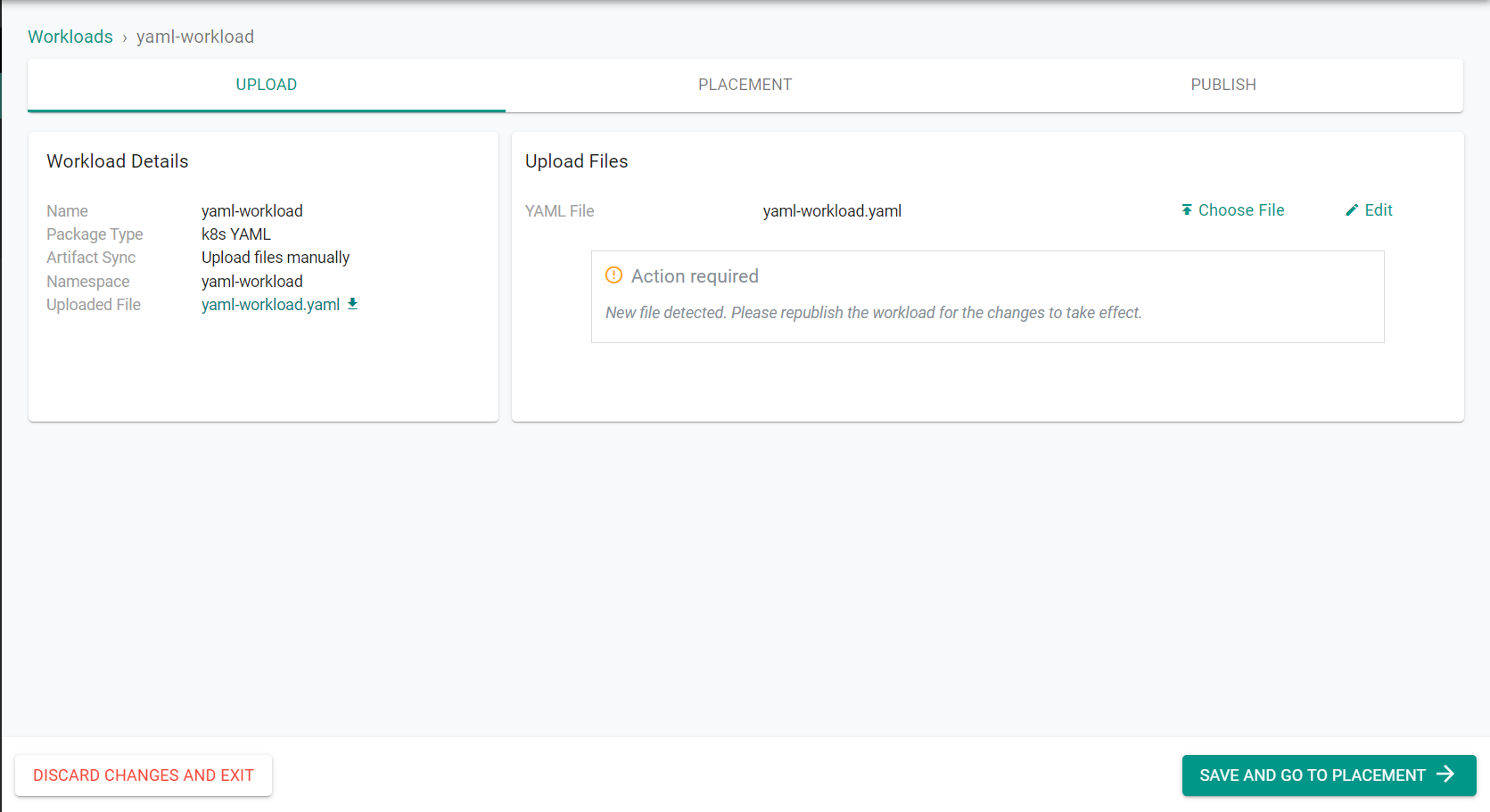The image showcases a user interface screen titled "Workloads," focusing on a specific workload named "Yamal workload." The screen is divided into various sections such as "Upload," "Placement," and "Publish," with the "Upload" section prominently highlighted in green.

In the "Upload" section, detailed workload information is displayed. Key details include the workload name, "Yamal workload," the package type "K8s Yamal," and the artifact synchronization method, which is "upload files manually." The namespace is also identified as "Yamal workload." Additionally, an uploaded file named "Yamal workload.yamal" is listed with a downward-facing arrow beside it, indicating the option to download the file.

Below the section for uploading files, the same "Yamal workload.yamal" file appears, accompanied by options to "Choose File" and "Edit." A prominent message with an orange exclamation mark indicates "Action Required." The message alerts users that a new file has been detected and prompts them to republish the workload for the changes to take effect.

At the bottom of the screen, two buttons are visible: a "Discard Changes and Exit" button in red text and a "Save and Go to Placement" button in green with a forward-facing arrow. The overall design is rendered in mostly gray and black text, arranged in a rectangular layout typical of a web page interface.